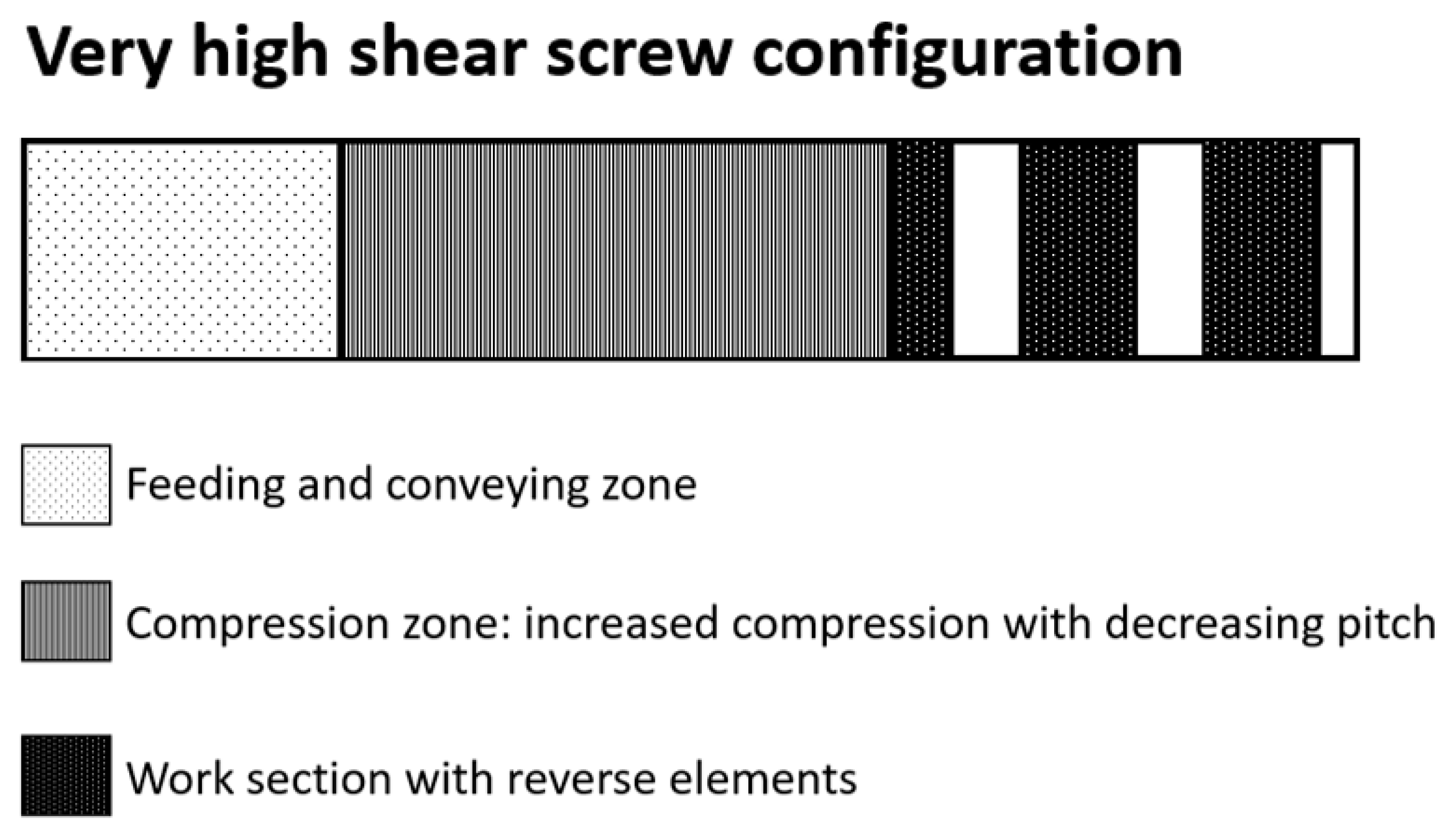The image depicts a technical illustration titled "Very High Shear Screw Configuration." The central feature is a horizontal rectangular bar segmented into various patterned sections. The first section is a white background with black polka dots, representing the feeding and conveying zone. The next, roughly double in length, has slender vertical black and white stripes, denoting the compression zone with increased compression and decreasing pitch. Following this is a narrower black section with white spots, signifying the work section with reverse elements. This pattern repeats with a plain white strip, another black section with white dots, a narrow white section, another black section with white dots, and finally a small white strip. The entire diagram is outlined in black. Below the bar, a comprehensive legend clarifies the meaning of each pattern: the polka-dotted section as feeding and conveying zone, the pinstripe section as compression zone with increased compression and decreasing pitch, and the black with white dots as the work section with reverse elements.